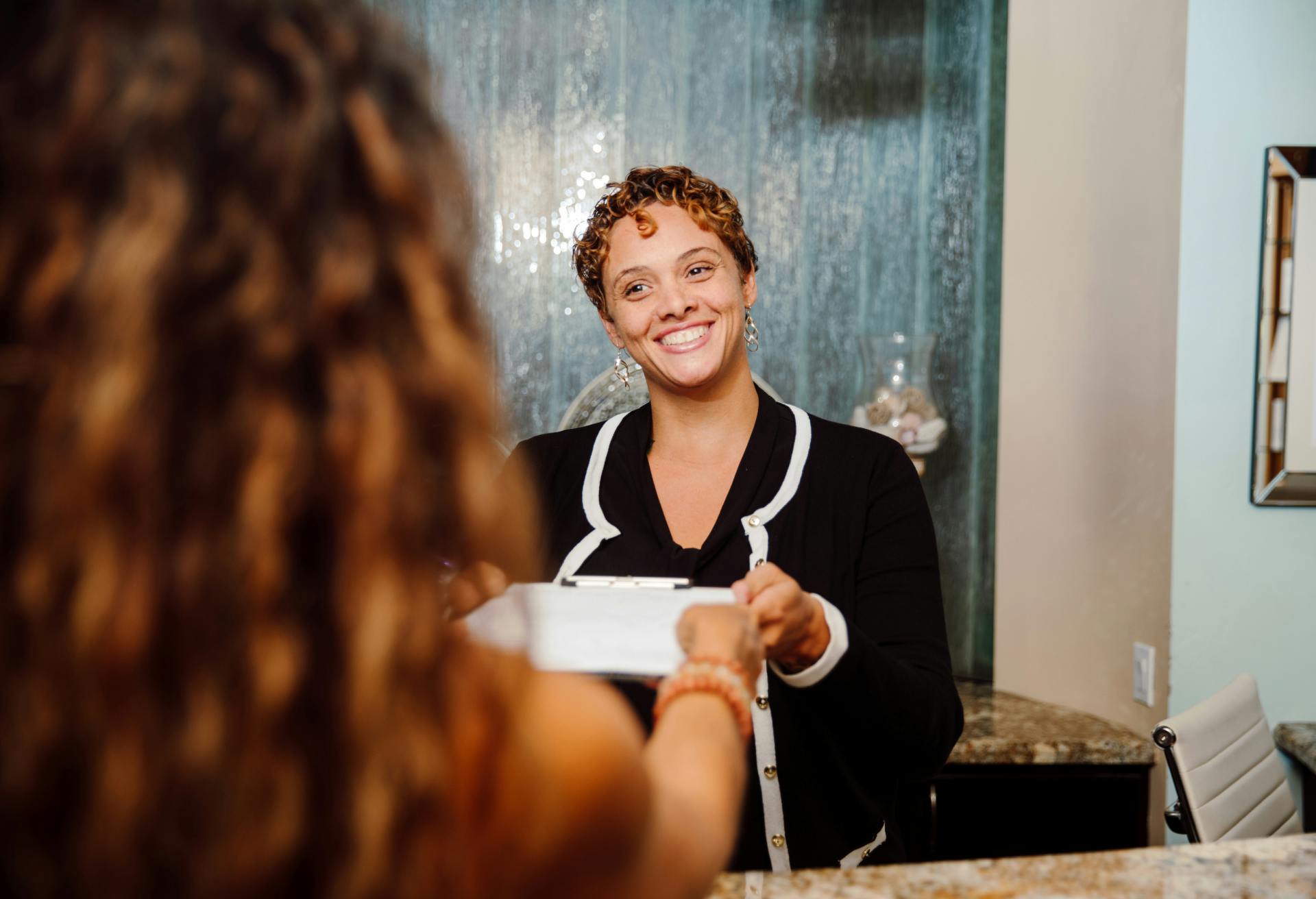In this photograph, a woman with short hair and golden earrings is seen smiling brightly while engaging in conversation with another woman who appears to be handing her a clipboard. The smiling woman is dressed in a dark cardigan sweater with white trim around the buttons and wrists. The setting suggests a professional interaction, likely related to a job interview, job offer, or contract discussion. One woman is positioned behind a marble-covered desk, potentially a credenza, while the other stands in front of her. The background features a shimmering, chromium-like wallpaper and a wall-mounted lamp that adds a subtle glow to the scene. Through an open doorway, an adjacent room with pale off-white walls, adorned with a painting and another chair, can be observed. The interaction between the two women, centered around the clipboard, suggests a formal transaction or business matter.